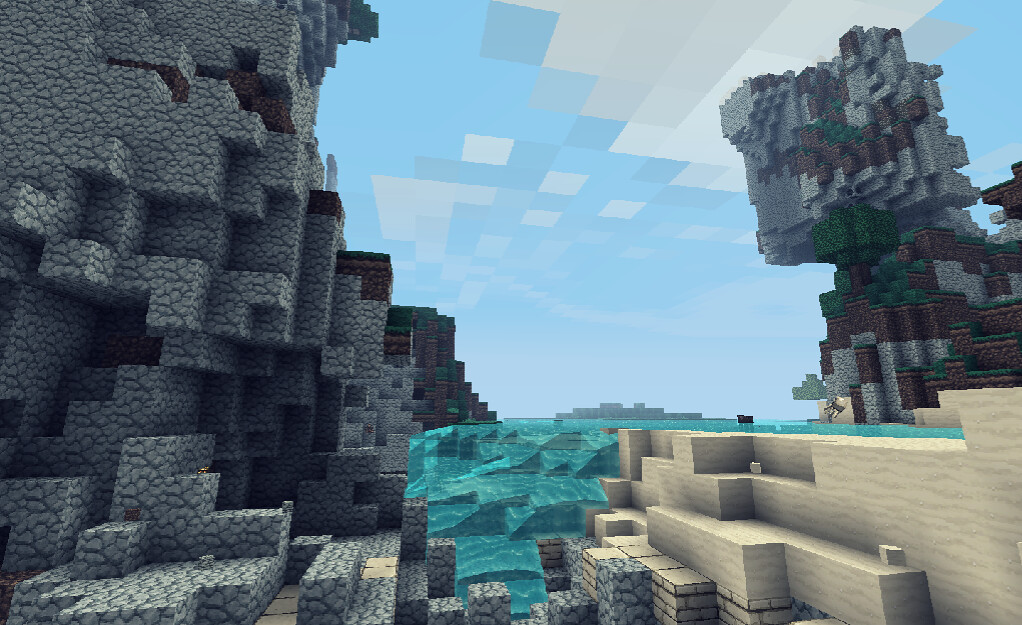This image, rendered with a video game aesthetic resembling Minecraft, showcases a vivid, cubistic landscape. On the left, there are stacked cubic formations with rocky textures, reaching high and filling much of the frame with shades of gray and interspersed brown, depicting a mountainous area. The center is dominated by aqua blue cubes with a water texture, creating a reflective, fluid appearance. To the right, there are light tan, sandy-textured cubes, forming a contrasting arid region, accented by streaks of darker beige. Smaller cubic elements appear as dark brown soil and green grass, with a tree formed from a brown trunk and green leaves. The sky above is composed of light blue and white cubic clouds, completing this intricate, voxel-style scene.